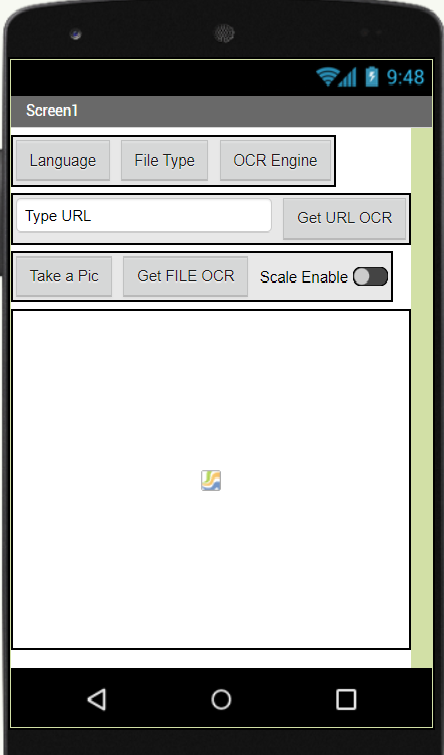This is a detailed, computer-generated image of a smartphone, depicted primarily in black with slightly fuzzy edges indicative of its digital origin. At the top of the phone screen, typical UI elements are displayed: a speaker and front-facing camera setup, a digital clock reading 9:48 on the right-hand side, alongside icons indicating full battery power, strong Wi-Fi connection, and full signal bars.

Below these elements, the interface features a text label reading "Screen One" in white lettering. Directly beneath the label, there are buttons labeled for "Language," "File Type," and "OCR Engine." Further down, a prominent white box invites the user to "Type Your URL," flanked on its right by a gray button with black text stating "Get URL OCR."

The next section contains another row of gray buttons labeled "Take a Pic," "Get File OCR," and a radio button for "Screen Enable," which can be toggled on and off. Central to the screen's lower half, a large white area is dominated by a generic placeholder image, represented by a square filled with yellow, blue, and green colors, symbolizing where a JPEG or picture would be displayed.

At the very bottom of the screen, typical browser navigation buttons are present: a "Go Back" button, a "Home Page" button, and a minimize button on the right-hand side. This meticulous representation showcases a blend of functional UI components designed for ease of use, all within the confines of a sleek, black smartphone.